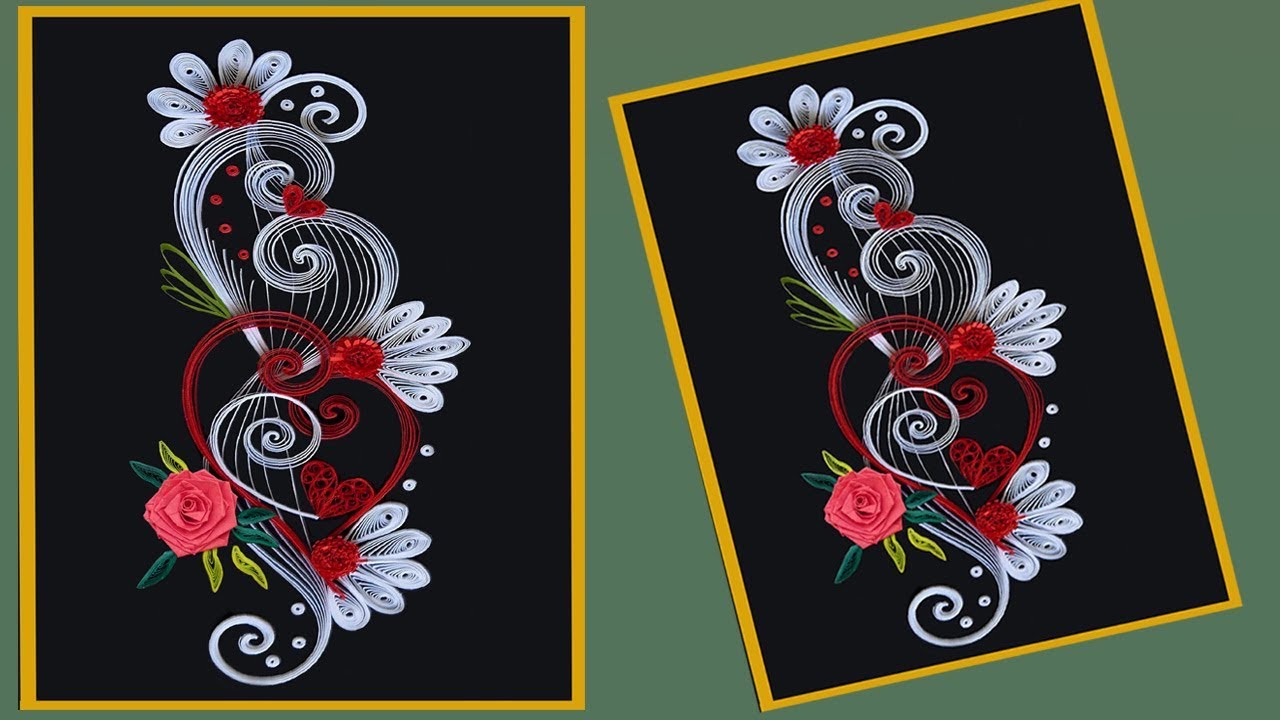The image showcases two identical square pieces of art, each adorned with a thin yellow border and set against a black background. The left piece is perfectly aligned vertically, while the right piece is tilted at an angle. Both squares feature detailed, thread-like designs intermingling various colors and elements. Dominating the center is an elegant white, g-clef-like swirl extending from the bottom to the top, adorned with a little white flower with a red center at the top. At the lower left, there's a prominent pink rose with green leaves. Scattered around the pieces, there are daisy-like white petals, small white dots, and intricate lines. The visuals depict a rich tapestry of threadwork, giving the art a textured, 3D appearance. Additionally, the background behind the squares is a forest green, enhancing the vivid colors and fine details of the floral and swirling patterns within the black interior of each square.